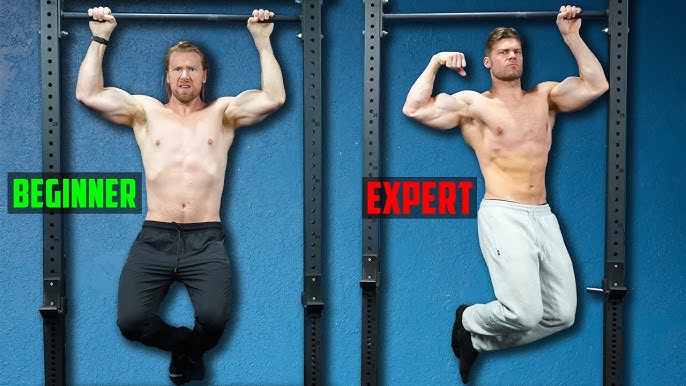The image depicts two shirtless, muscular Caucasian men performing pull-ups on a blue mat set against a blue wall with black metal frames. The setup includes two pull-up stations, each labeled to indicate different skill levels. On the left, the man labeled "Beginner" has blondish-brown hair and wears dark blue pants and shoes. He is struggling to perform a pull-up using both hands on the bar. In contrast, the man on the right, labeled "Expert," showcases his advanced strength by performing a one-handed pull-up while making a muscle with his free arm. He is wearing light gray or white pants and tennis shoes. The side-by-side comparison emphasizes the progress from beginner to expert in pull-up proficiency.